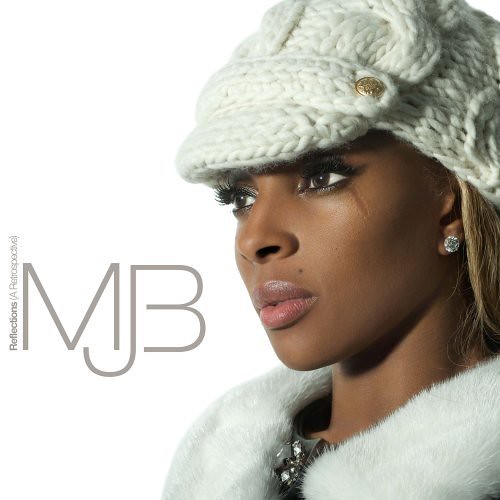The professional photograph, which appears to be an album cover, features Mary J. Blige against a white background. The left side of the image contains the text “Reflections Retrospect” in gray letters, followed by “MJB”, implying her initials. The close-up on the right side showcases Mary J. Blige adorned in a white knitted cap with a brim and a gold button. Only the left side of her face is visible, highlighting her striking dark green eyes accentuated by thick eyelashes and eyeliner. Her skin is clear except for a scar under her left eye, above her cheek. She has a mole above her full pink lips, and she wears a diamond stud earring in her left ear. Mary J. Blige is dressed in a luxurious white fur coat with diamond embellishments, underneath which she appears to be wearing a black or gray top with gemstone buttons.